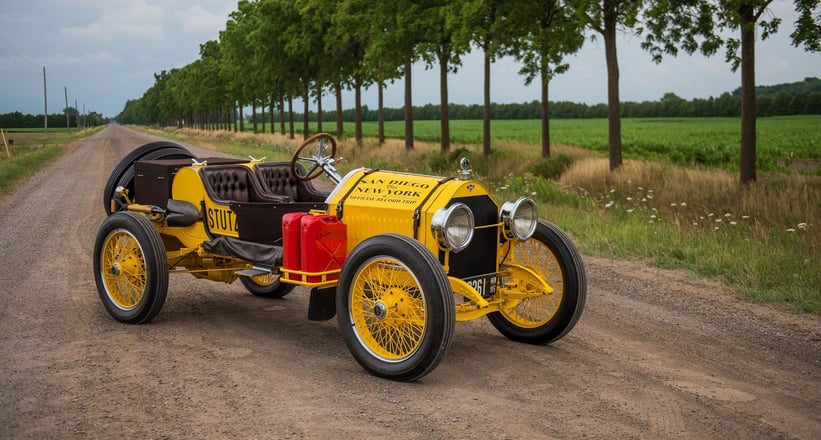The image captures a detailed view of a vintage yellow automobile, with a design reminiscent of old racing or touring vehicles. The car, positioned centrally and diagonally, features thin, large wheels with black rubber tires and yellow rims, akin to oversized bicycle wheels with intricate metal spokes. Prominent are its two large silver headlights and black grills at the front. The vehicle, devoid of a roof, showcases two black leather seats and a brown steering wheel. Notably, there are two red jerry cans attached to the side in a special holder, hinting at extended travel needs. Additionally, there's a shovel strapped to one side and two spare tires mounted at the back. The setting features a wide, brown dirt road flanked by upright trees with green leaves, and a grassy field dotted with small white flowers on the right side of the image. The sky appears blue, enhancing the scene's vintage charm.